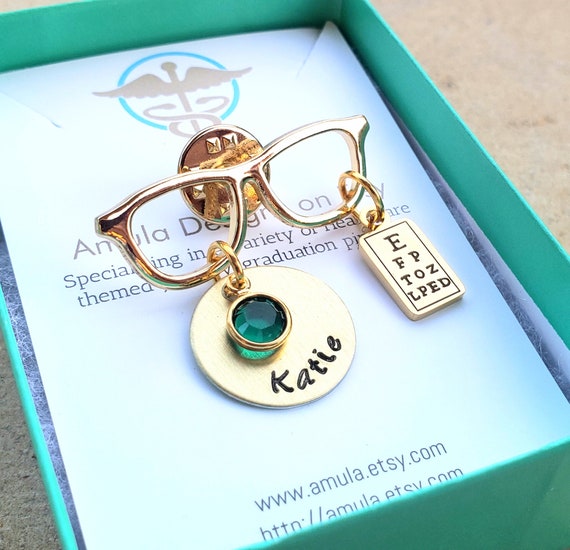This photograph showcases a detailed, close-up view of a gold pin shaped like a pair of glasses, displayed within an open green box with a white interior. The gold glasses feature intricate details with each lens replaced by a metal hoop. Hanging from the left hoop is a round trinket with a smaller charm inlaid with a green stone, while the right hoop holds a rectangular charm that emulates an eye chart with black letters decreasing in size from E to D. The words "Katie" are inscribed on a blue tag, adding a personalized touch. Above the glasses on the box is a medical symbol, featuring wings and a caduceus (a staff with two snakes entwined). Partially obscured text is present behind the glasses, making it difficult to decipher fully, but the bottom of the box clearly displays the website "www.amula.etsy.com." The box itself is nestled on brown paper, highlighting its rich teal-green color. This combination of elements suggests a carefully crafted, medically-themed jewelry piece possibly related to optical professions or personalized gifts.